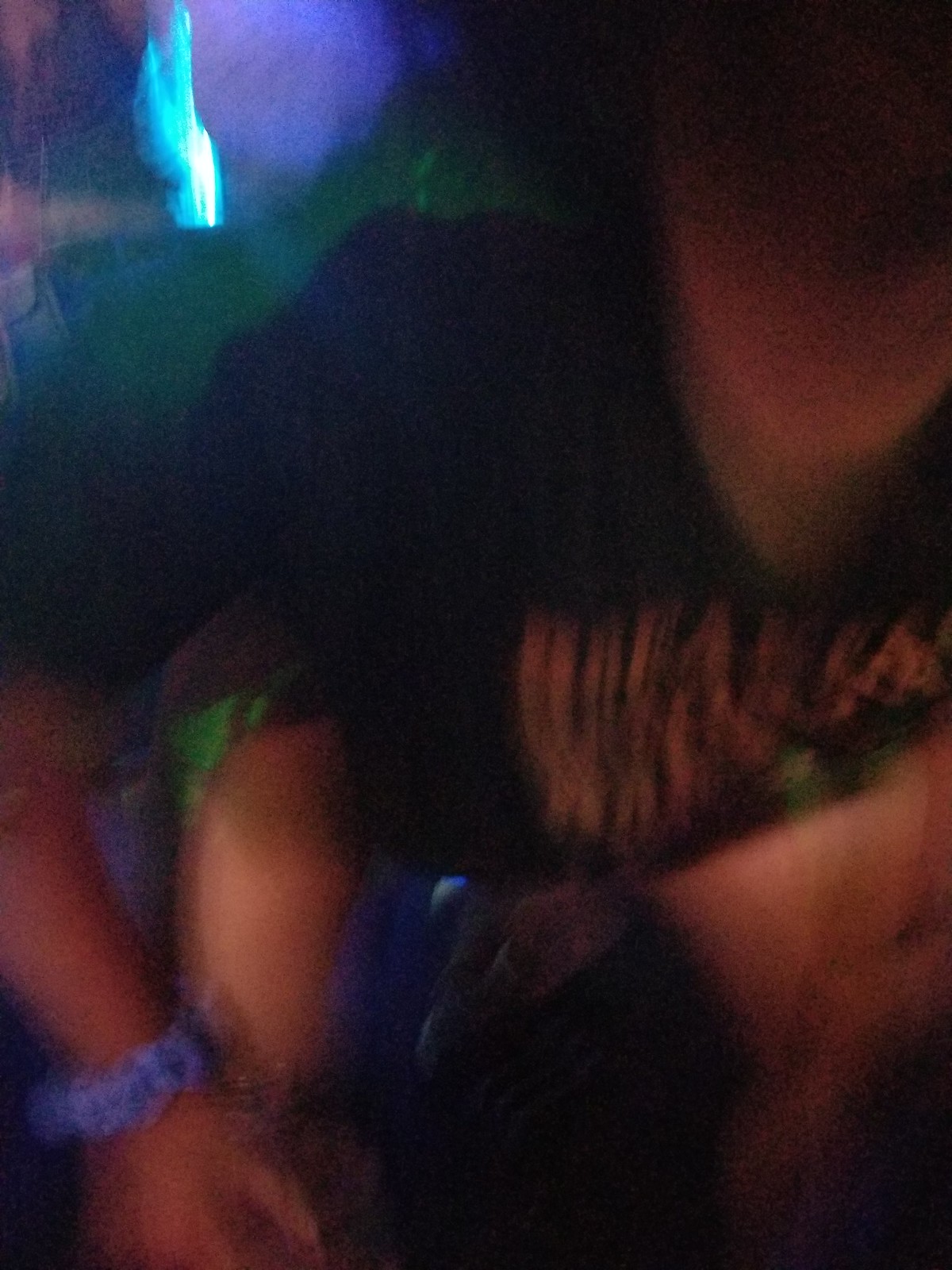In this extremely blurry, low-resolution color photograph, a woman is visible, looking directly at the camera. She is wearing a black t-shirt with illegible red or orange text and a green bracelet on her arm. The photo is so out of focus that her face is obscured, with only her chin slightly discernible. Beside her, part of another person's right arm is visible, adorned with what appears to be a purple or blue scrunchie. The vague background reveals indistinct blue and green lighting, possibly from a flame or a lamp, although the poor quality of the image makes it impossible to determine the exact source. The overall scene is chaotic and unclear, resembling something taken accidentally.